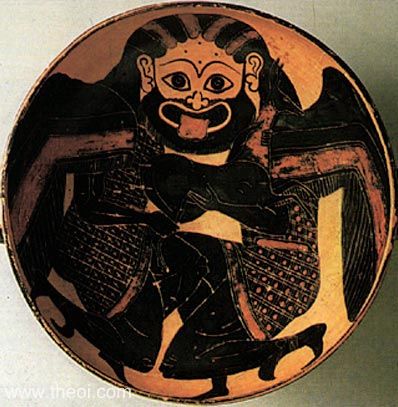This detailed, close-up picture showcases an enigmatic round object, possibly a coin or pottery dish, set against a gray background. The object, appearing old and weathered, features a complex design rendered primarily in black, white, and light brown hues. The central motif is a fusion of two figures with black legs and arms, adorned in black dresses with white patterns. Each figure has black and white wings extending from their backs and reaches out towards the other. Their heads mesh together to form a singular face with a large, black beard, big black eyes, and an expressive, protruding tongue. The hair is depicted with black and white streaks, and there are four dots in a diamond shape on the forehead. The edge of the object has a black border, contrasting with the gold-toned interior. The overall appearance is cartoonish yet detailed, evoking an image of some ancient, mythological artifact.